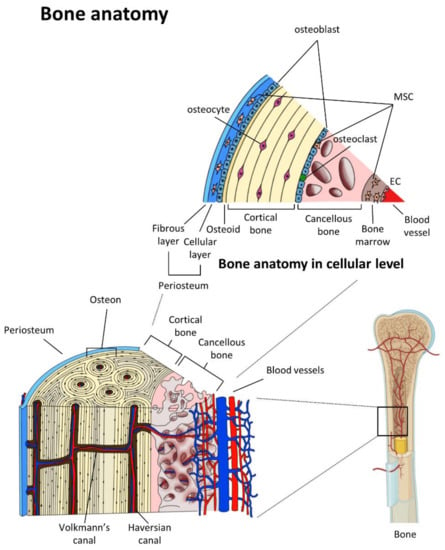The image displays detailed diagrams of bone anatomy, with a bold heading at the top that reads "Bone Anatomy." There are three primary diagrams. The main diagram on the lower right illustrates a bone, likely a femur, colored in shades of brown with red veins running through its top portion. This bone has a cross-section revealing a yellow cylinder that transitions into a peach-colored inner cylinder.

Two other zoomed-in diagrams expand on this bone structure. One zoomed-in section, highlighted by a square, magnifies the bone's interior, showing a thin light blue exterior layer and a yellow body with swirling patterns and red veins. This section also displays blood vessels in red and blue, leading into a porous area. Labeled parts in this diagram include periosteum, osteon, cortical bone, cancellous bone, Haversian canal, and Volkmann's canal.

The second close-up, located at the top right, presents a simplified view labeled with cellular components and structures such as osteocyte, osteoblast, MSC, osteoclast, EC, blood vessel, bone marrow, osteoid, cellular layer, and fibrous layer. Text surrounding these illustrations highlights anatomical terms and emphasizes the bone’s cellular composition, including periosteum and the detailed vascular and cellular structures within the bone.